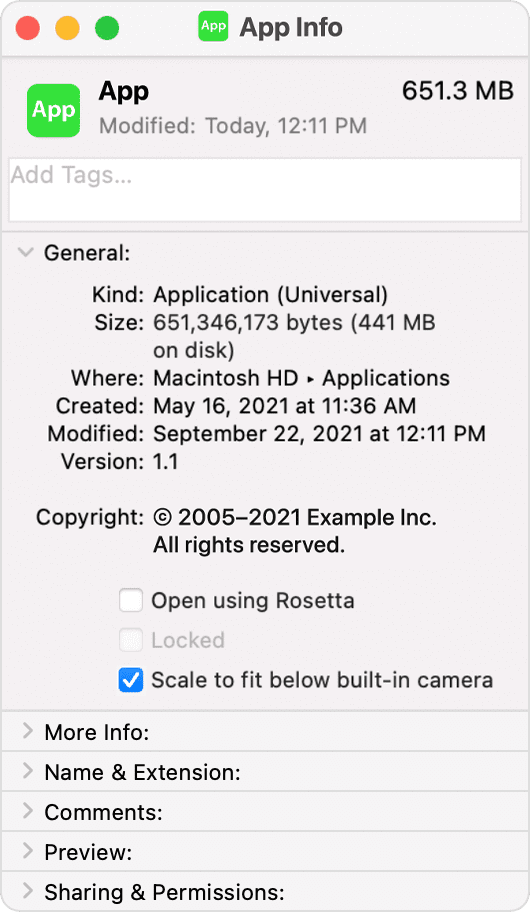A smartphone screenshot displays detailed application information in a structured format. At the top, "App Info" is prominently displayed. On the left side, there are three circular indicators: a red dot, a yellow dot, and a green dot. Adjacent to these, the application's logo is shown as a green square with "app" centered within.

Below the header, the logo is repeated, with the word "app" directly below it. The modification date is listed as "12-11pm," and to the right of this, the file size is noted as "651.3 megabytes." Beneath this, there is a tag entry box for adding labels.

In the main body of the screenshot, a drop-down arrow reveals detailed app information:
- **General Information:**
  - **Kind:** Application (Universal)
  - **Size:** 651,346,173 bytes (441 megabytes on disk)
  - **Location:** Macintosh HD > Applications
  - **Created:** May 16th, 2021 at 11:36 AM
  - **Modified:** September 22nd, 2021 at 12:11 PM
  - **Version:** 1.1
  - **Copyright:** 2005-2021, Example Inc., All rights reserved.

Several checkboxes are available for user interaction:
- **Open using Rosetta**
- **Locked**
- **Scale to fit below built-in camera** (checked)

Additional expandable options include:
- **More info**
- **Name and extension**
- **Comments**
- **Preview**
- **Sharing and permissions**

This screenshot provides a comprehensive view of the application's properties and available settings for the user.